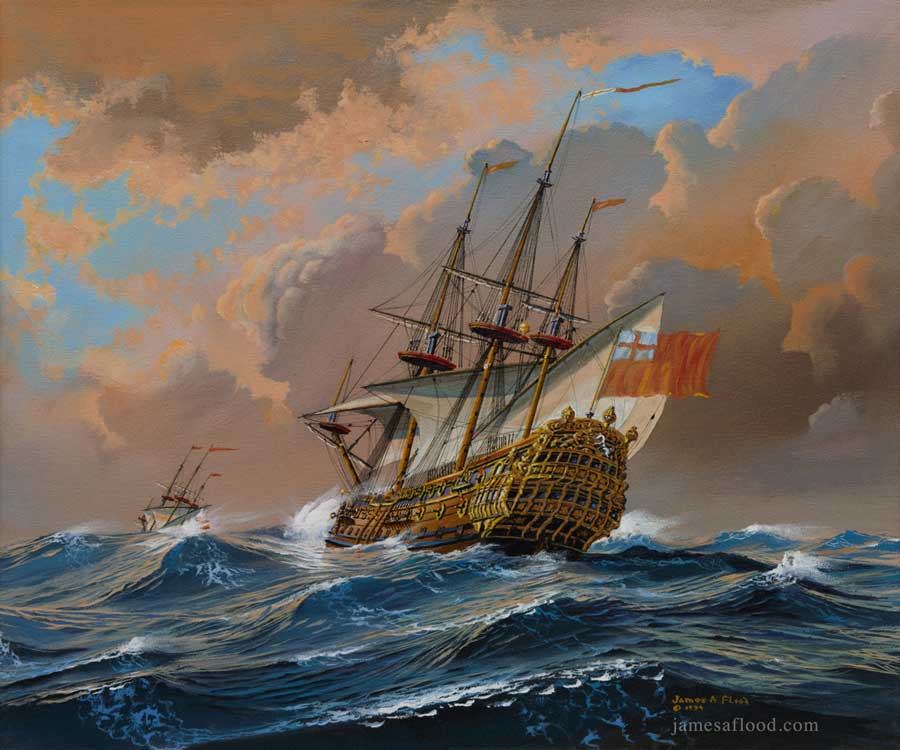This painting vividly captures a dramatic maritime scene featuring two ships navigating through rough, dark blue ocean waters under a turbulent sky. The sky covers the top two-thirds of the painting and is an ominous mix of gray and orange clouds, with glimpses of blue peeking through, suggesting an impending storm or a dramatic sunset. Below, the ocean is depicted in dark blue hues, with white-tipped waves fiercely crashing.

Dominating the center of the painting is a large, brownish galleon with gold trims, slightly tilted to the right due to the tumultuous waves. It has three prominent masts with sails, some of which are furled, and atop the masts are little flags. An orange flag with a white square and orange cross flutters at the back end of the ship. In the distance to the left, another smaller ship is barely visible, also flying similar flags.

In the bottom right corner of the painting, the artist's name, James A. Flood, is written in yellow, with the website jamesaflood.com beneath it in white letters. The detailed rendering of the ships, the foreboding sky, and the turbulent sea combine to create a powerful and evocative maritime scene.